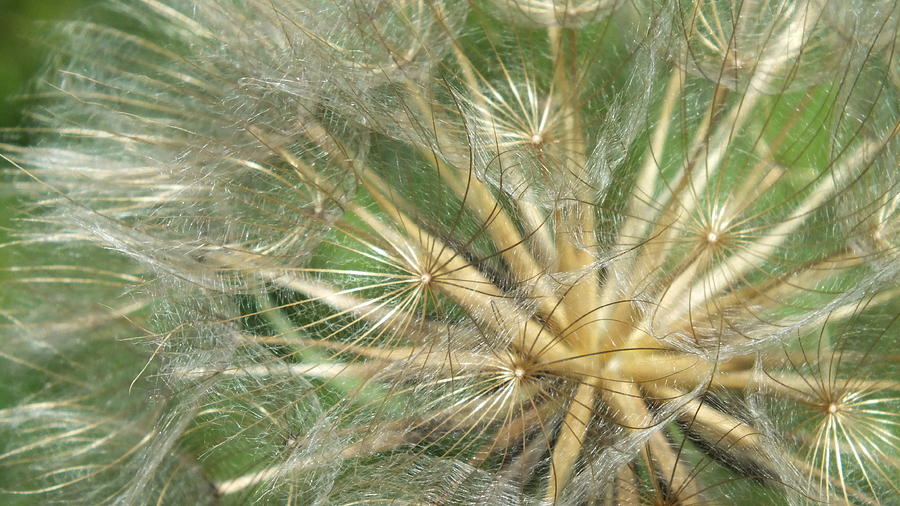This close-up image captures the intricate details of a plant resembling a dandelion in its seed stage. The photo, likely taken for educational purposes, focuses on the plant's structure, showcasing small, fibrous-like flowers that appear ready to disperse. The plant features multiple brownish stems, each culminating in a delicate, almost umbrella-shaped array of thin, silky threads. These threads interweave to form a web-like structure, reminiscent of spun glass or spider webs. The background blends various shades of green, suggesting a natural outdoor setting, with darker greens toward the center, emphasizing the plant's central anatomy. The overall effect is a stunning zoomed-in view that highlights the delicate and ephemeral beauty of the seed dispersal phase, with the white, lacy petals seemingly caught in a gentle breeze, poised to drift away.